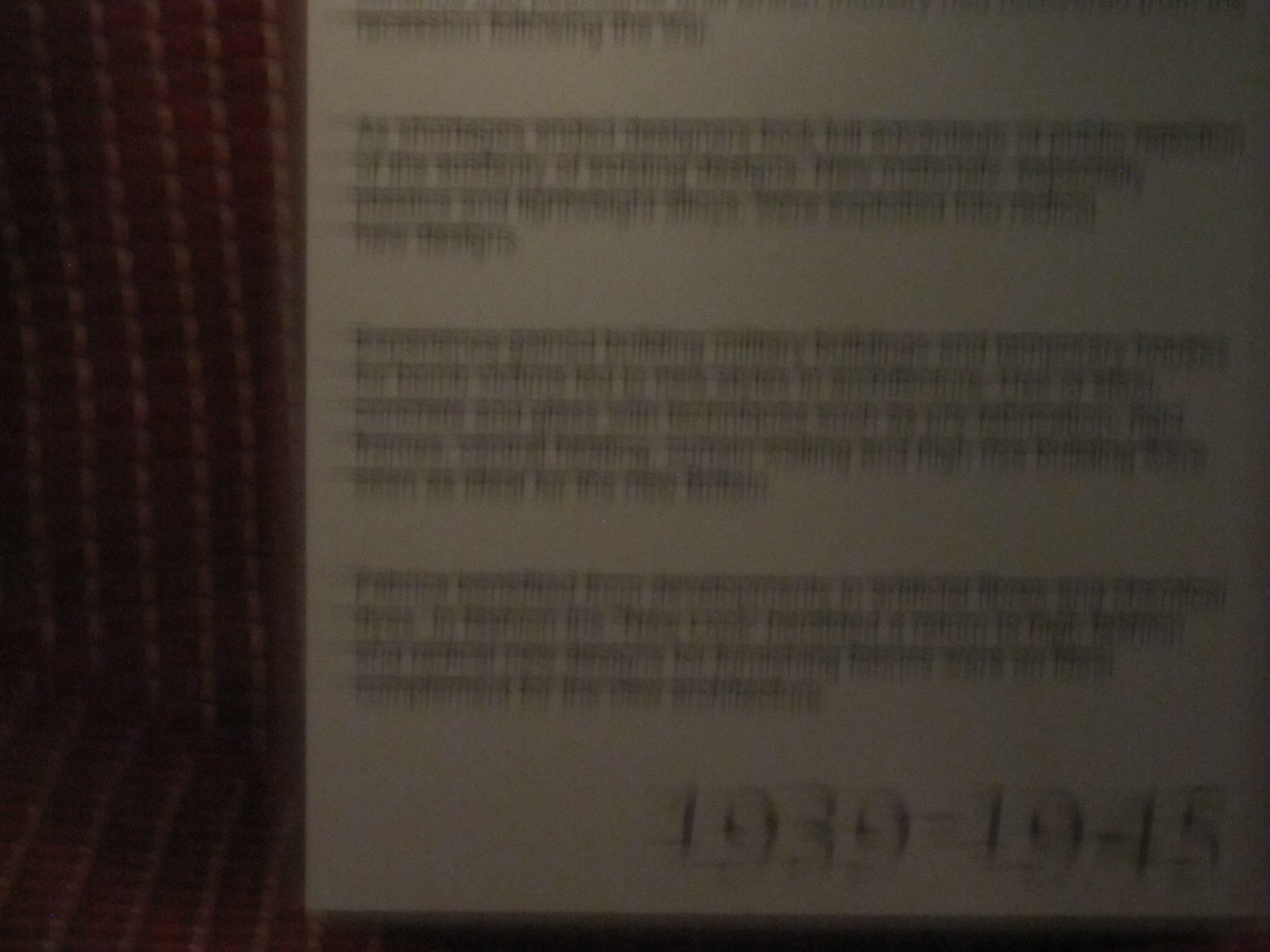The image depicts a photograph of a white piece of paper, which appears to contain a typed letter. The text on the paper is printed in black ink and consists of three paragraphs. Although the specific content of the letter is indiscernible due to blurriness, the bottom of the paper prominently features the dates "1939-1945." At the top of the paper, there is a single line of text, which could either be a heading or the beginning of the first paragraph. The exact words and details within the letter remain unclear due to the image's lack of clarity.